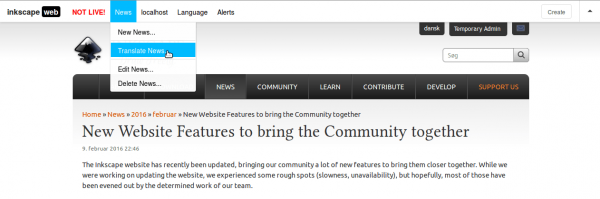A screenshot of a homepage is displayed, showcasing a new website feature aimed at fostering community engagement. The details on the page are difficult to decipher due to the small and unclear text. A menu is highlighted, distinguished by a gray background and a light blue selector, although the specific menu items are illegible. The overall purpose of the site or the page remains unclear, as the image does not provide sufficient detail to understand its full context or functionality.